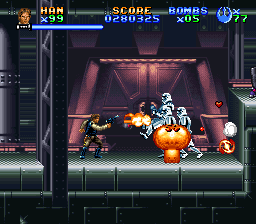This is a detailed screenshot of a retro-style side-scrolling video game, reminiscent of an old Star Wars game. The scene features Han Solo, armed with a blaster, engaged in combat with two stormtroopers. One stormtrooper is oddly perched on what seems like an orange pumpkin-like seat, adding a quirky element to the industrial setting. Han Solo is depicted on the upper left corner along with statistics: his name followed by "X-99" indicating lives, a score of 0280325, and a count of "bombs X-05". Another icon next to a trident-like symbol displays the number 77. The industrial background has a purplish hue with steel elements, including dark gray flooring with light gray highlights and a pair of closed purple steel doors. The ground is dark black steel, complemented by steel support beams. The scene is further heightened by visual effects, including fireballs emanating from Han Solo's gun and small mushroom-shaped explosions, contributing to the vibrancy of the colors despite the game's older style.